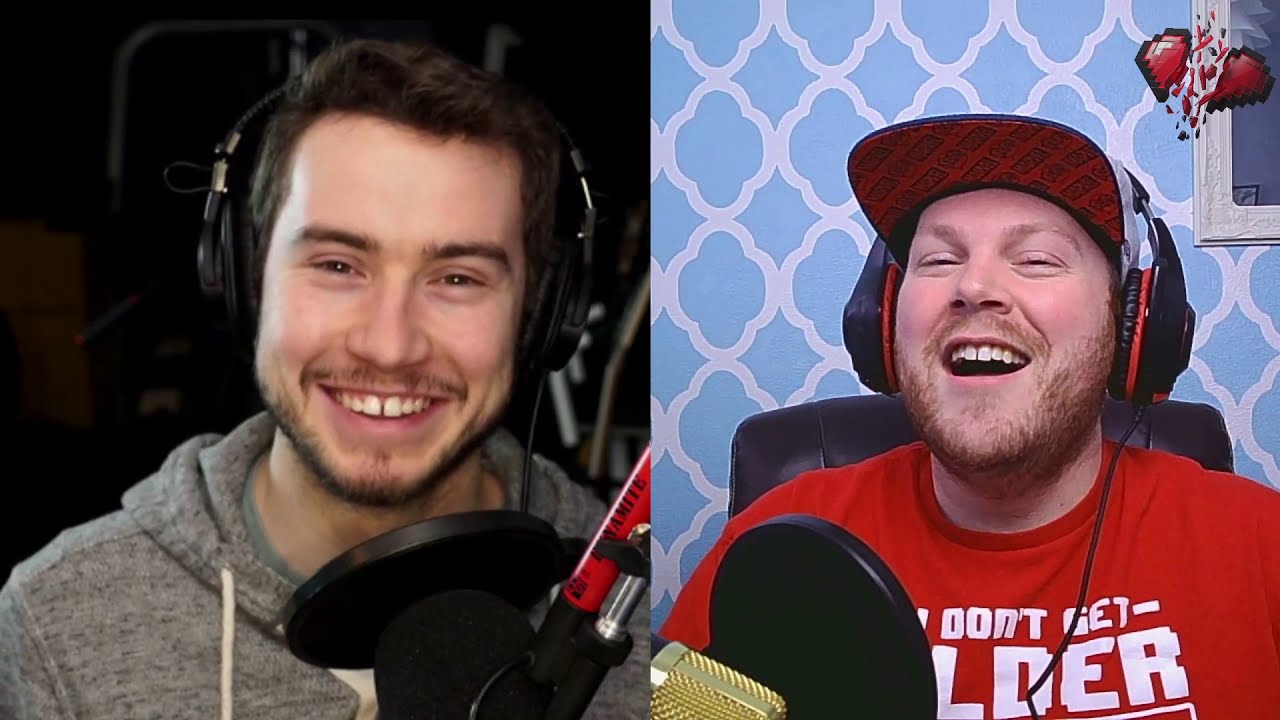In this image, two men are pictured side by side, seemingly in a podcast setting, both smiling and possibly laughing. The man on the left, who has short black hair and some facial hair, is wearing a gray hoodie and headphones. He is in front of a microphone and a dark background, smiling directly at the camera. The man on the right, also wearing headphones, has lighter hair and facial hair. He is adorned in a red baseball cap and a red shirt with partially visible text reading "Don't get [L-D-E-R]." The background behind him features a blue-on-blue design with a CGI-style broken heart emblem in the upper right corner. The colors in the image include various shades of black, white, blue, red, gray, gold, and a touch of purple. Both microphones are large, black, and circular, hinting at a lively discussion, likely during a podcast episode.